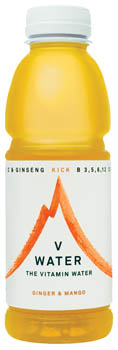This image displays a single-serve, translucent yellow bottle of "Vee Water," a type of enhanced vitamin water, set against a plain white background. The bottle features a white lid and a white label that wraps around its middle. Prominently displayed on the label is an orange logo resembling a mountain with two peaks, giving it a dynamic, brush-stroke appearance. The main text on the label, written in green and black, identifies the drink as "Vee Water, the vitamin water," and specifies the flavor as ginger and mango. Additional text includes terms like "ginseng" and "rich," alongside some nutritional details that are partially obscured by the bottle’s curvature. Accents in the same orange color as the logo further decorate the label.